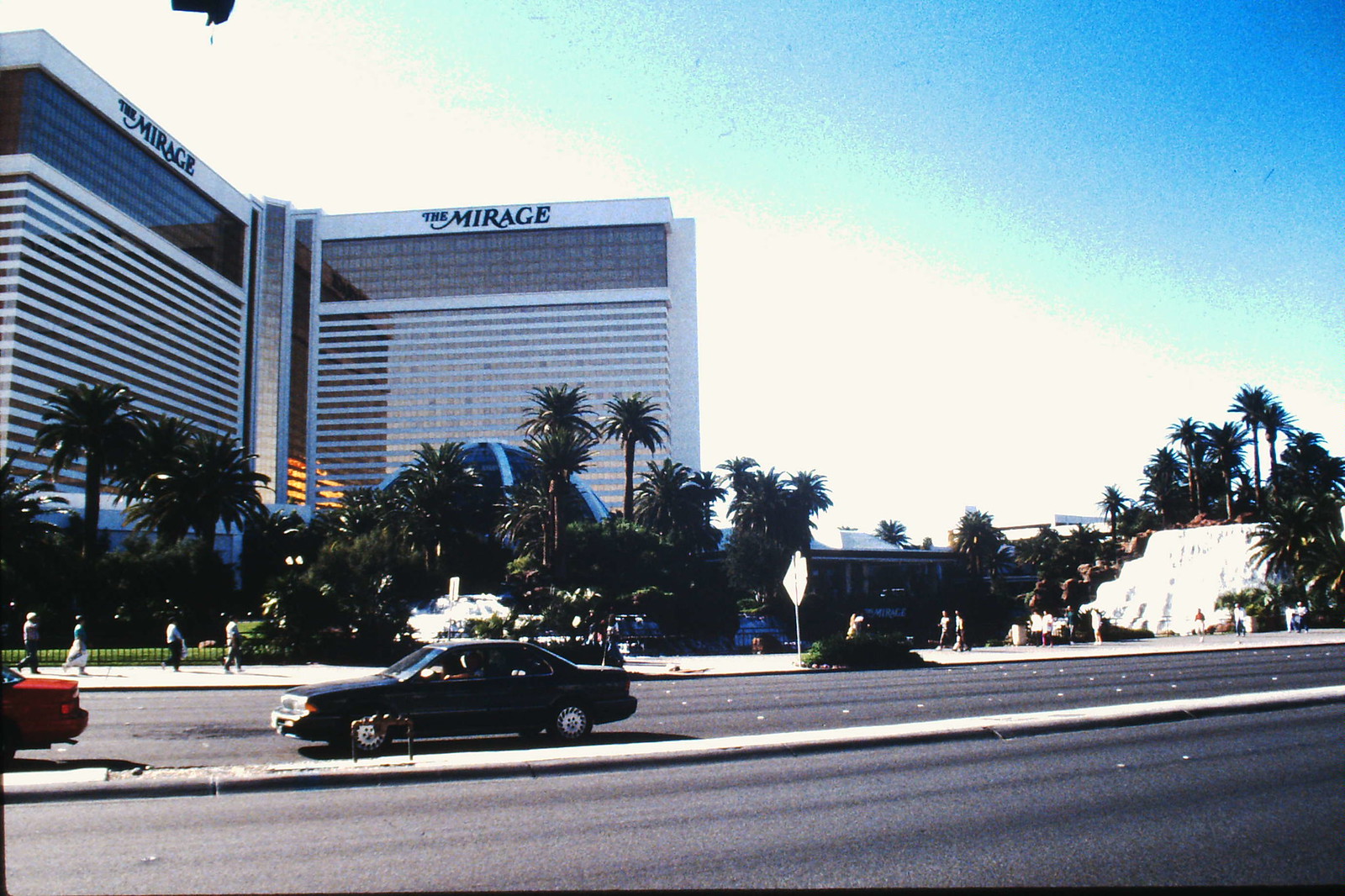This image captures an old photograph, likely taken in Las Vegas, featuring the Mirage Hotel and Casino as its centerpiece. The Mirage building dominates the left side of the frame, showcasing its distinctive architecture that resembles an open book, with its two wings extending perpendicularly. The building is a large white complex with prominent "The Mirage" signs on both wings. Below the building, a line of palm trees flanks the street, along with what appears to be artificial waterfalls on the right side. The foreground presents a long asphalt road with a black car and a red car driving towards the left. On the left side of the road, people are walking along a sidewalk, which continues on the right side of the image. The photo is bathed in bright sunlight under a clear blue sky, with some vintage photo characteristics indicating it might have been taken with an old film camera or through an editing filter. The image captures the vibrant, yet timeless, essence of this iconic Las Vegas location.